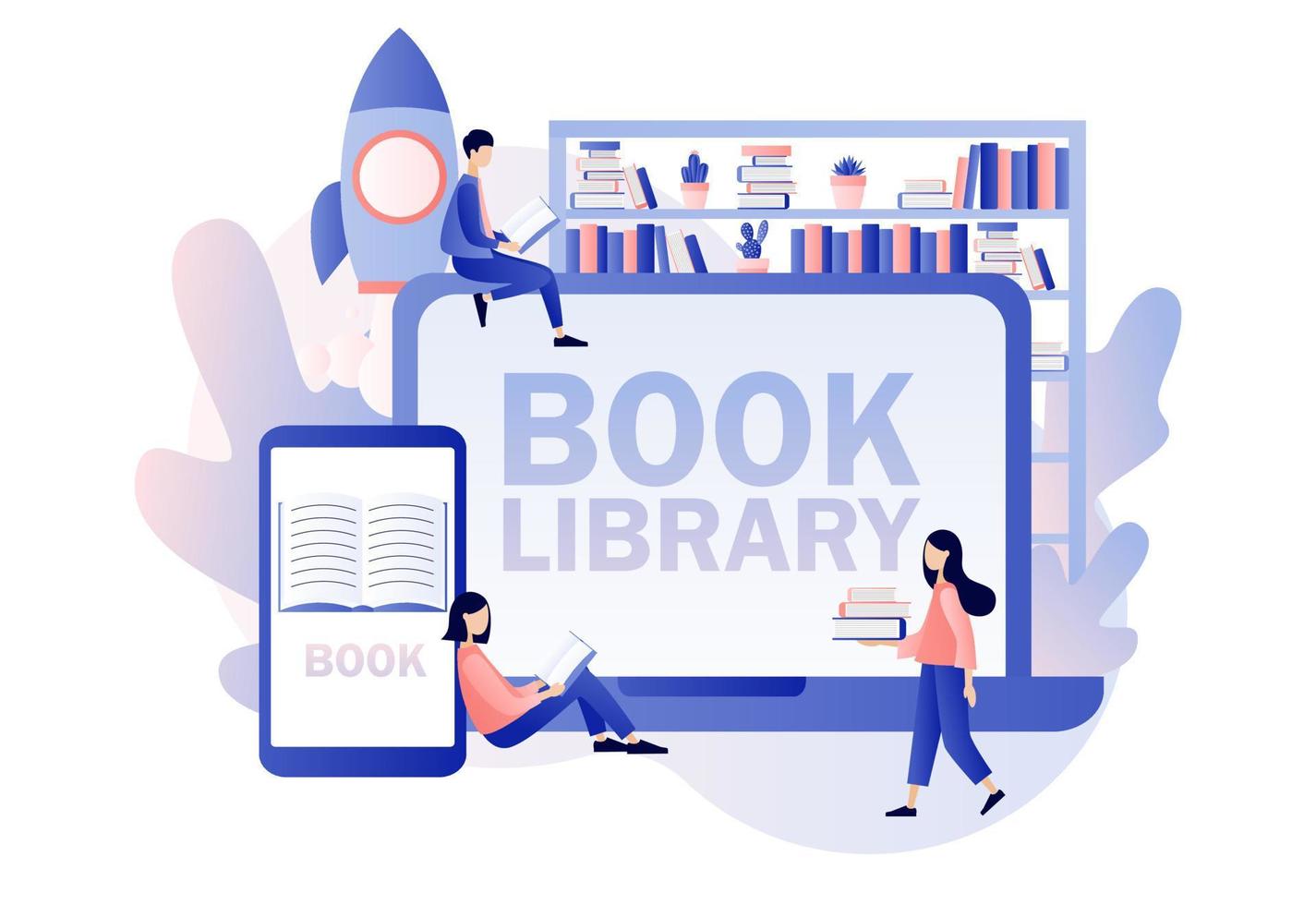In this cartoon image, a dynamic and colorful scene shows three faceless female characters and an animated background. Centrally featured is a large laptop with a white screen displaying the words "BOOK LIBRARY" in light blue. One of the females is sitting atop this laptop, engrossed in her book, clad in all blue with black hair and shoes. Another female, in a pink shirt and blue pants with black hair and shoes, leans casually against a nearby tall, rectangular object resembling a phone or tablet. This device has an open book icon and the word "BOOK" in caps on its white screen. To the right, yet another female wearing similar attire walks while balancing three books—one blue and two pink.

The backdrop consists of five bookshelves outlined in shades of blue, adorned with a mix of blue and pink books and plants, including two cacti. At the top left corner, there is an eye-catching rocket ship in blue and orange hues, complete with a red-circled white window. Additionally, light blue blotches decorate both the left and right sides of the image, contributing to the playful and whimsical atmosphere.